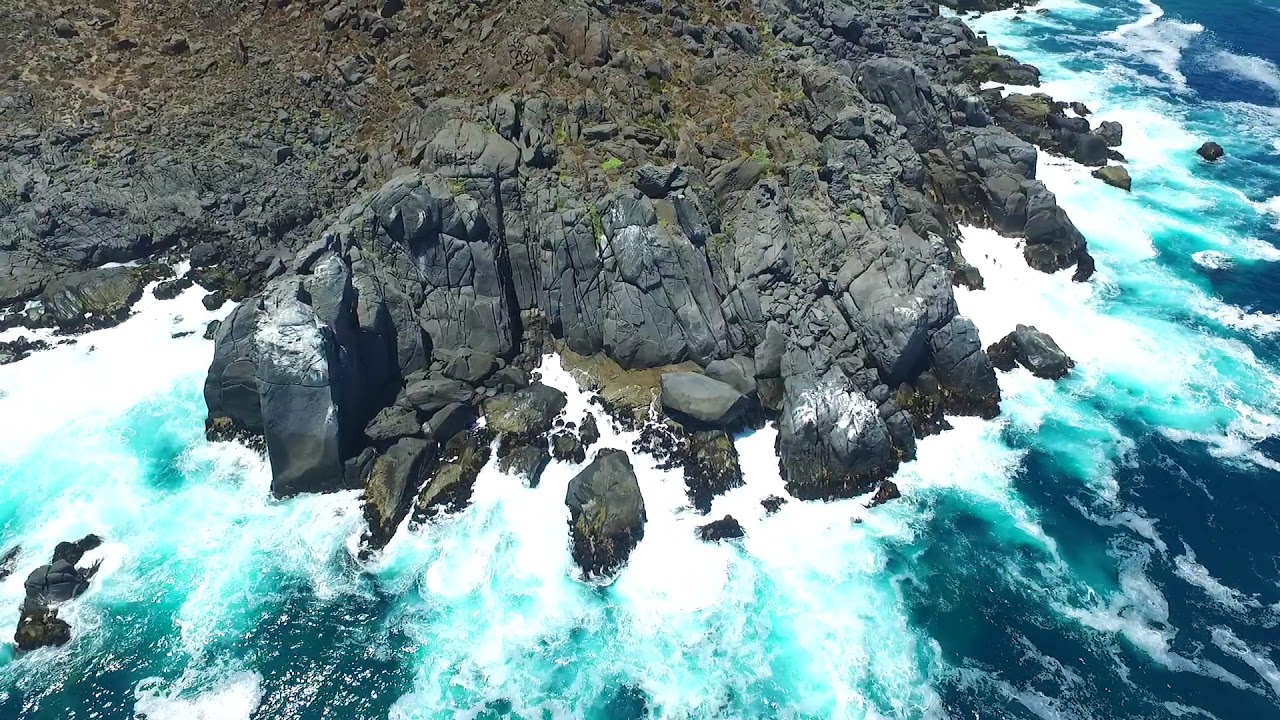This aerial photograph, likely captured by a drone from a height of about 70-80 feet, showcases a stunning coastal scene where rugged cliffs meet an active and foamy body of water, possibly an ocean or sea. The top half, especially the upper quarter, of the image is dominated by mossy-colored, green and tan rocky formations which resemble cliffs. These cliffs, centered in the photo, are interspersed with patches of grass and vegetation, creating a mix of green and tan shades. The gray rocky cliff face contrasts strikingly with the vivid blue, clear waters below. The waves are forcefully crashing against the cliffs, forming beautiful white foam, and the bright sunlight enhances the clarity of the scene. The image lacks animals, people, man-made structures, and any textual elements. The dynamic interaction between the cliffs and the frothy waters offers a mesmerizing view of nature's raw beauty.